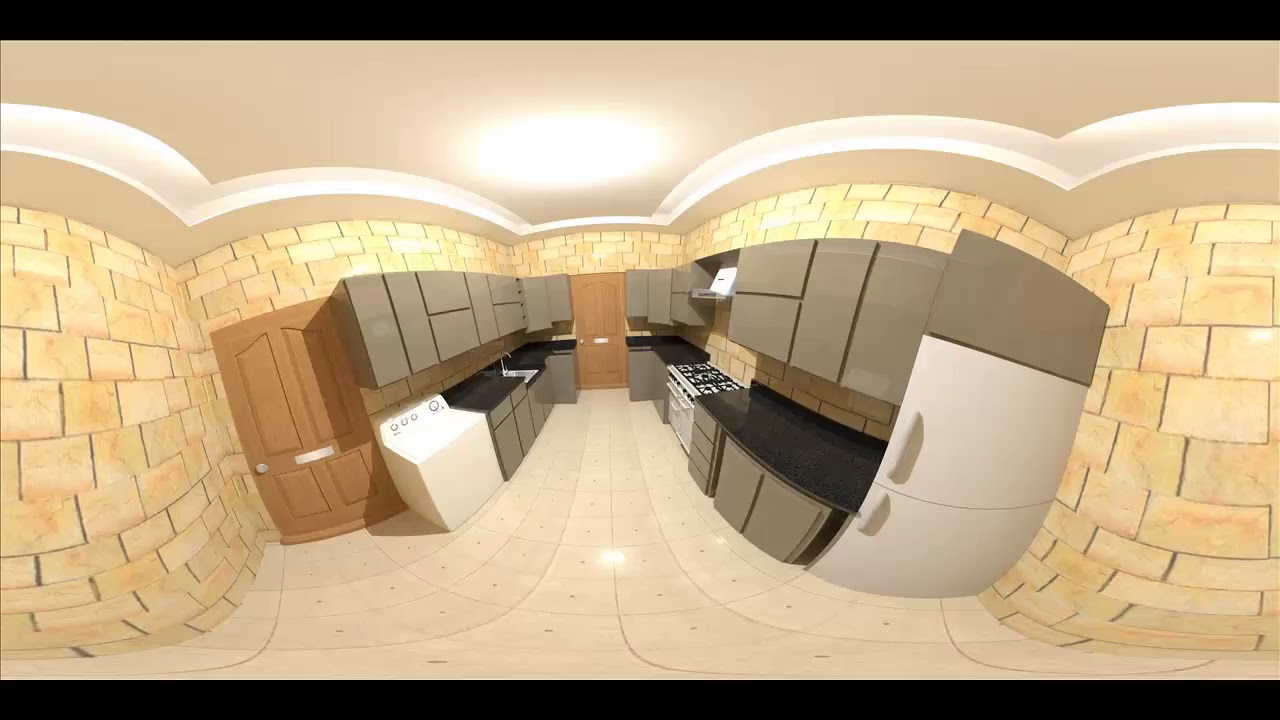The image depicts a modern galley kitchen with beige tile walls and light brown cabinetry. The ceiling features elegant curved molding that stretches across the top, contributing to the room's aesthetic appeal. The right side of the kitchen hosts a white refrigerator, white stove, and a white sink, all set against light brown cupboards. Below the cupboards, the countertops appear to be a deep gray granite, adding a sophisticated touch. The floor consists of tiles with subtle spots, enhancing the space's texture. At the far end of the kitchen, a door between cabinets leads outside, while another door to the right provides access to the pantry. The kitchen exudes a sleek, modern vibe with its cohesive color scheme and curved architectural details.